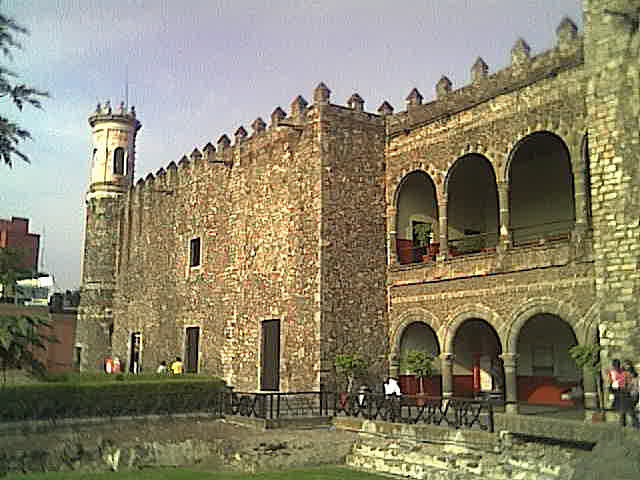The photograph depicts an exterior view of an ancient stone castle, likely of medieval origin, dominated by gray, irregularly stacked stones that emphasize its age and weathered charm. The castle stands at least two stories tall with a walkable third level, crowned with crenellations resembling childlike drawings of sharp spikes. To the left, a cylindrical watchtower, adorned with statues, rises majestically where the wall terminates.

On the right side of the image, the castle features an array of elegant arches forming a patio and balcony, suggesting a grandeur that overlooks a distant body of water. The arches, colored white at the top and red at the bottom, span two stories, creating a series of corridors on each level. Below these arches, three equidistant rectangular doors punctuate the wall, accompanied by a solitary window positioned centrally.

Foreground elements include a slightly pixelated and artifact-laden view of the courtyard, hinting at the photo's old age and possible compression. The courtyard is accentuated by a three-step staircase near the bottom right that leads to the castle's entrance, flanked by potted plants and bordered by a lush green hedge. Further to the right, a wrought iron fence extends from the hedge, adding a touch of elegance.

Groups of people are dispersed around the photograph: two or three individuals can be seen on the far right, and two more wander towards the left along a path adjacent to the hedge. The sky overhead appears overcast with bluish-gray clouds, possibly pregnant with rain, adding a moody and historical ambiance to the scene.